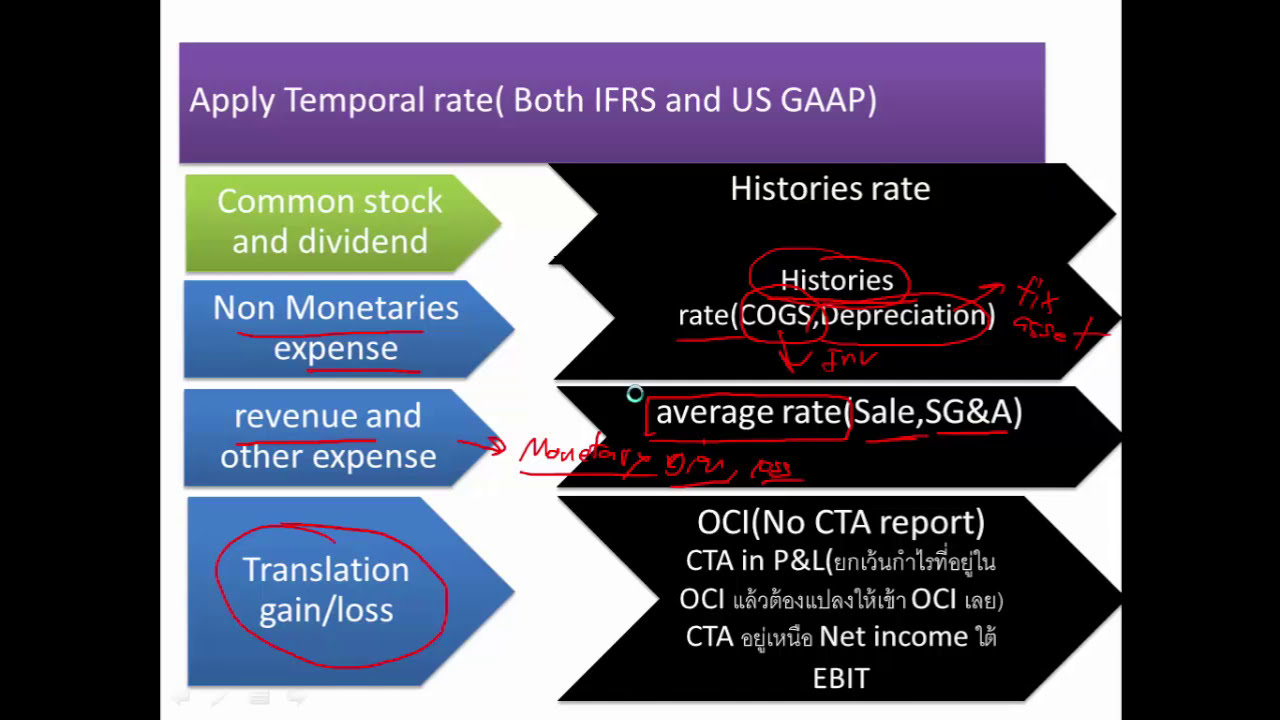The image is a detailed, color-coded page from an accountant's guidebook, framed by thick black borders on both sides. At the top center, a purple block with white text states, "Apply temporal rate (both IFRS and USGAAP)." Below, there are five distinct lines with blocks in different colors containing various accounting terms and principles. 

The left column starts with a green block that says "Common stock and dividend" and features an arrow pointing right. Following this is a blue block with "Non-monetary expense," another blue block with "Revenue and other expense," and a bottom blue block stating "Translation gain/loss," all with arrows pointing right. These elements are interspersed with red circles and annotations highlighting important points, such as "notes" and corrections like "fix, CS set" and "INV."

On the right, black blocks with white text list terms such as "History's rate," "COGS depreciation," "Average rate," "Sales, SG&A," with further details in the bottom blocks, including "OCI (no CTA report)," "Net income," and "EBIT." The terms "history's rate" and "History's rate" also appear multiple times, emphasizing their importance, with additional red-pencil marks suggesting corrections and notes.

Overall, the page is visually clear with a structured layout emphasizing various accounting rules and terms through distinct colors and annotations.